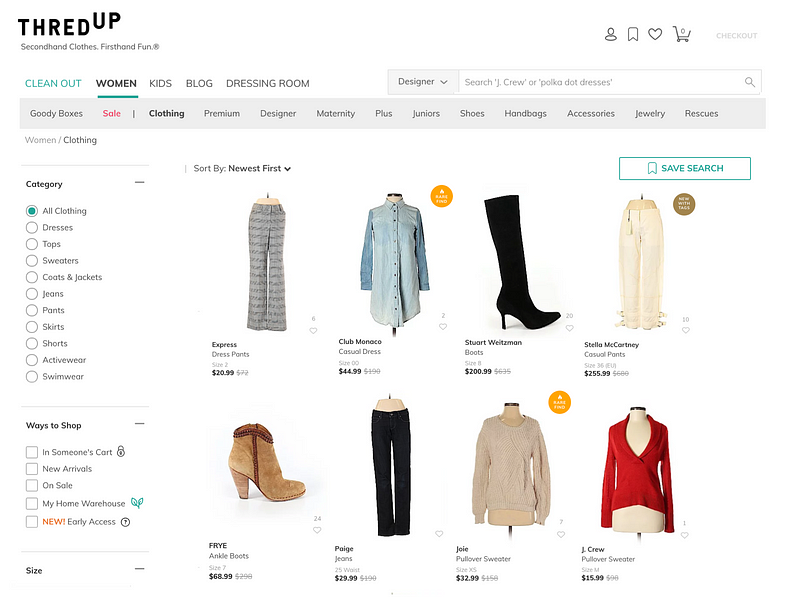This screenshot captures a user's shopping experience on the ThredUp website. The interface features a clean, white background. On the right-hand side at the very top, we see that the user's shopping cart is currently empty, indicated by a count of zero. The left side of the screen displays various shopping categories, with the user having selected the "All Clothing" category. 

The central section showcases an assortment of clothing items available for purchase. These include:
- A pair of pants from Express,
- A long blue shirt,
- Tall black boots,
- A red low-cut top,
- Short suede boots,
- A pair of jeans,
- A white sweater,
- White pants with a ruffled design.

At the bottom of the screen, there are options labeled "Ways to Shop," which likely offer different browsing methods or filters. On the right-hand side, the user can save their search or click on the heart-shaped "love" button at the top to add items to a favorites list, allowing for easier access to preferred products.